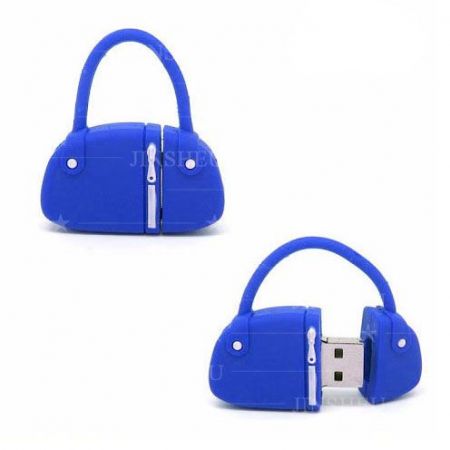The photograph showcases a USB device designed to resemble a stylish purse, set against a white background. The device is predominantly a royal blue color with distinctive features that enhance its purse-like appearance. The upper left section of the image features the USB device in its closed form, highlighting a blue, quarter-circle body with a prominent white zipper-like design, adorned with two white circular attachments at the base of its handles. These handles, made of blue plastic, connect the two parts of the device, adding to its purse illusion. The bottom right section reveals the USB device open, displaying the metallic silver tip that can be plugged into a computer. This clever design allows the device to function as a USB stick while maintaining an attractive appearance that mimics a small handbag when not in use.